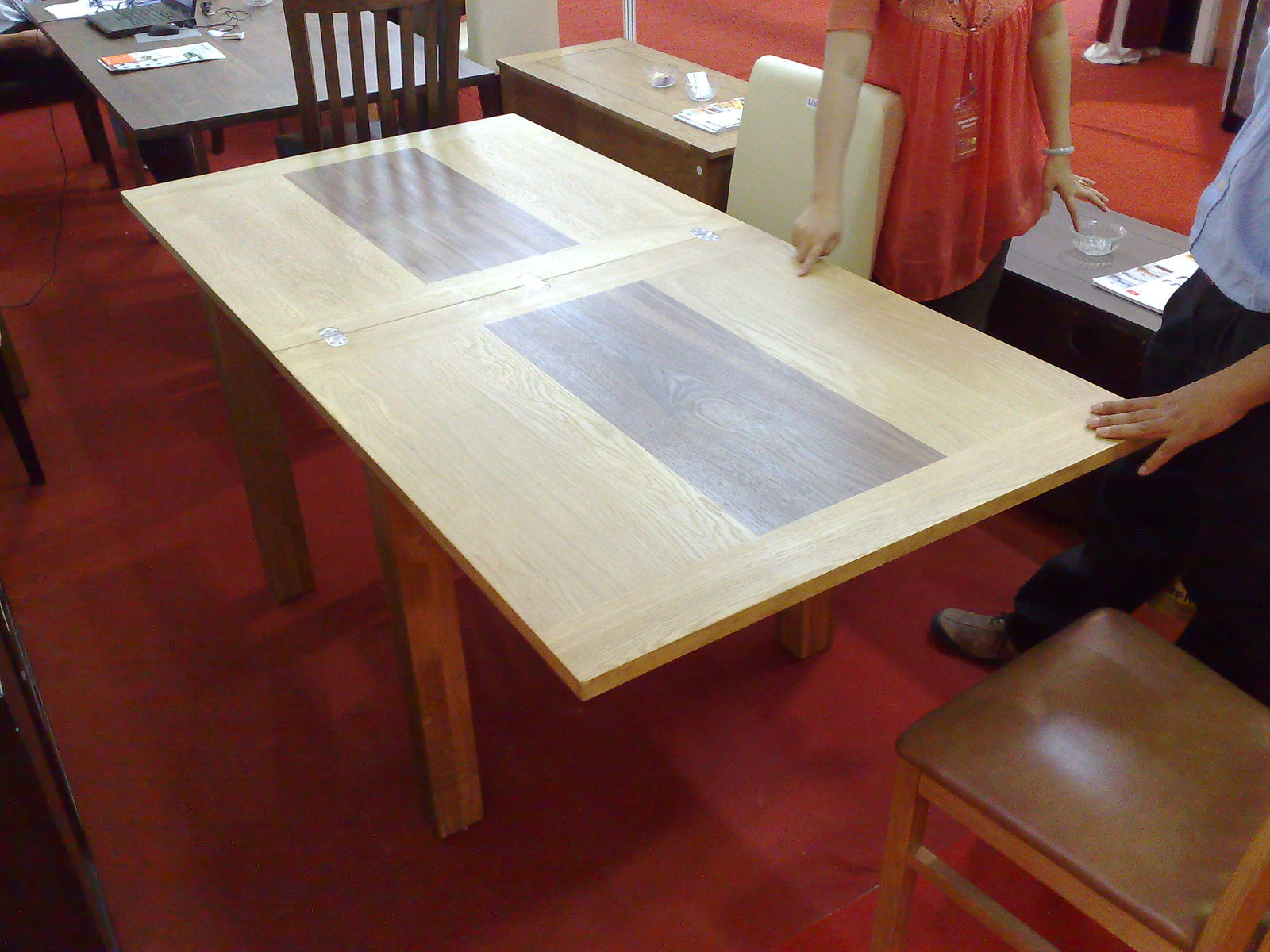In this detailed colour photograph, we see a scene that appears to be set in a furniture showroom with a rich red carpeted floor. Dominating the center of the image is a light brown rectangular folding table featuring a distinctive dark, greyish-brown strip running down the middle. This table's configuration suggests it might be composed of two square tables placed together. The table has wooden legs and visible metal hinges, enhancing its folding design.

Two individuals are closely examining the table. To the right, a well-dressed man, visible from shoulders down, is wearing a light blue button-up shirt, black trousers, and brown shoes; his left hand is resting on the table. Adjacent to him, a woman stands just left of center, identifiable by her reddish or pinkish blouse with a silver bracelet adorning her wrist. She has a slightly sheer, flowing shirt and dark pants. Her right hand is pointing or touching the surface of the table.

Surrounding the main table, there are several other pieces of furniture. To the immediate left of the table, a dark brown chair with a brown cushion and light brown legs is partially visible. Behind the woman is another table, darker in color, which holds a laptop and some promotional material. Additionally, there's a smaller light brown table stand to the right and a black table further in the background. A cushioned chair with a creamy grey back is pulled under the table in the background, contributing to the layered composition of the showroom setting.

The overall backdrop reveals hints of other tables and desks, one distinctly black and another brown, contributing to the bustling yet organized atmosphere of the showroom. A mirror or reflective surface behind the central figures adds depth, capturing partial reflections of the elements within the scene. The photograph captures a moment of interaction and consideration, highlighting the detailed features and textures of the furniture on display.